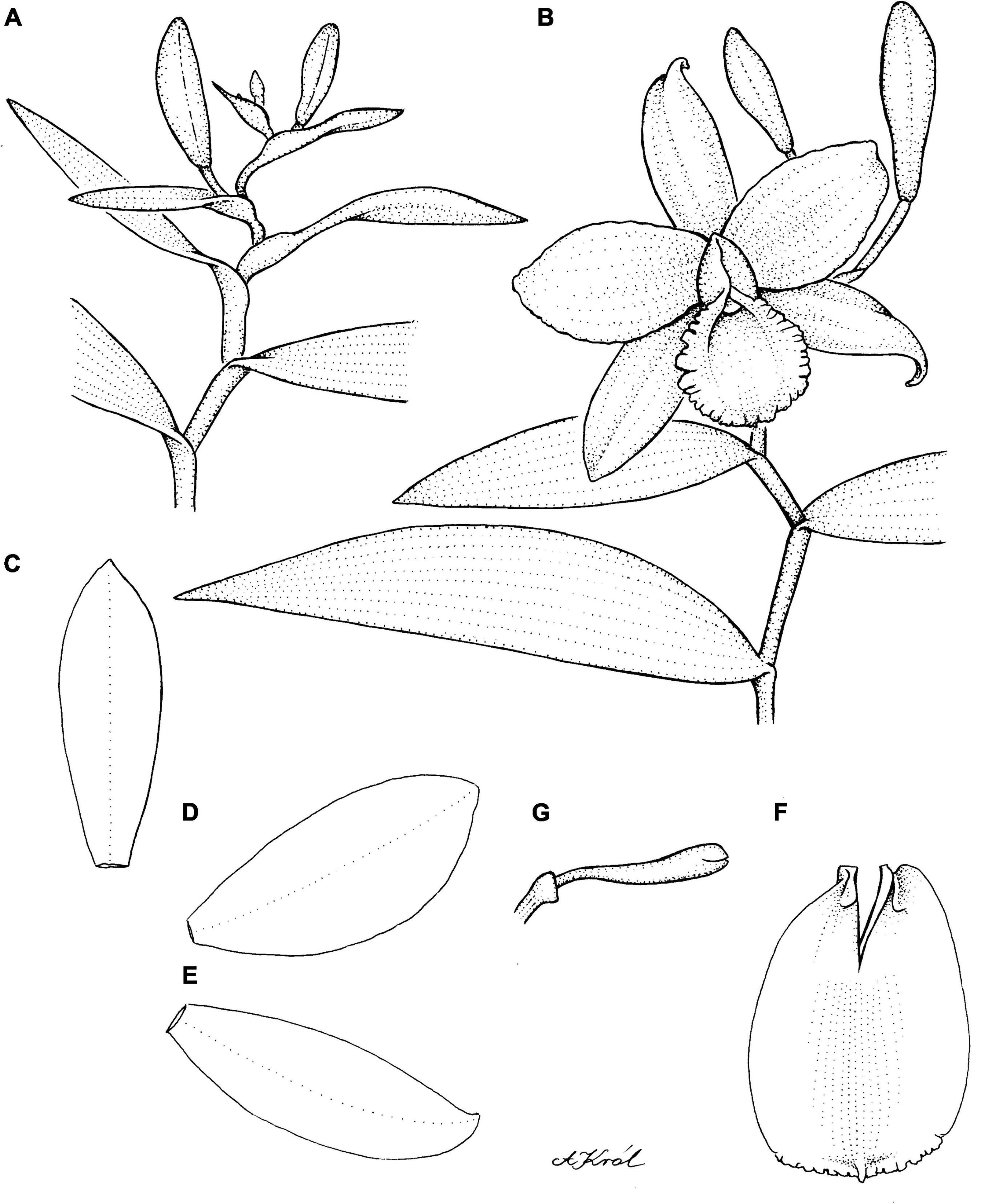This detailed illustration showcases various parts of a specific plant, most likely an orchid, labeled from A through G. The depiction includes a full-bodied view of the plant highlighted in section A, which accurately captures the foliage and stems. Section B offers a close-up of the stereotypical flower petals, intricately dotted to enhance detail. Sections C, D, and E each portray individual leaves of the plant, shown with simple outline drawings that lack significant depth or shading but are connected by dotted lines. Section F illustrates a closed flower bud resembling a tulip, while section G presents another part of the plant, possibly an unopened flower bud. The illustration is completed with the artist's signature at the bottom, adding a personal touch to the detailed botanical study.